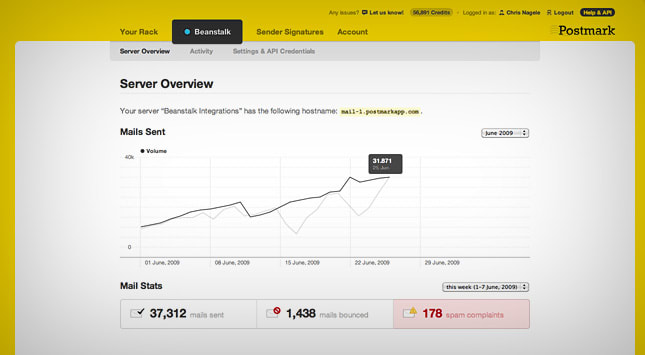The image is a screenshot of a computer dashboard, specifically a web page with a mustard-yellow border. At the top right-hand corner, the page features a small menu in black font reading, "Any issues?" with a chat icon labeled "Let us know." The page shows the user logged in as Chris Negele, with a bubble displaying a certain amount of credits, alongside a logout button. A black circle with the words "Help" and "API" in yellow font is also visible. 

The main navigation bar, situated above the page content, includes tabs labeled "Your Rack," "Beanstalk," "Sender Signatures," and "Account." The "Beanstalk" tab is highlighted in black font with a blue button next to it. The body of the page is primarily white, enclosed by a gray border with a header section indicating "Server Overview," "Activity and Settings," and "API Credentials," all in gray font except for "Server Overview," which is highlighted in black.

In the main content area, "Server Overview" is prominently displayed in black font. The central feature of this section is a graph with black, white, and gray lines titled "Mail Sent." Below the graph, mail statistics are showcased in a box with red font, stating "37,312 mails sent," "1,438 mails bounced," and "178 spam complaints."